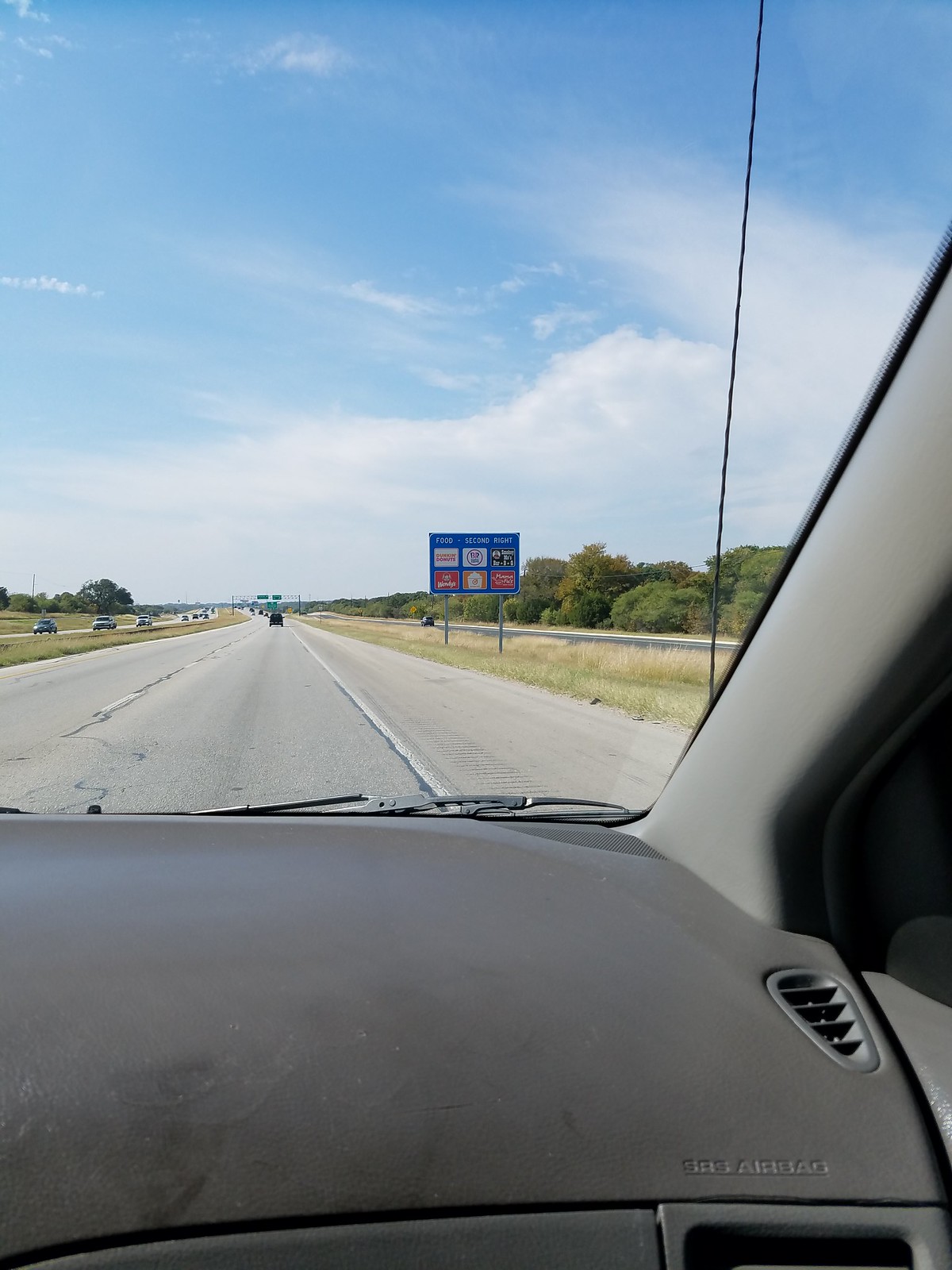The photograph, taken from the passenger side inside a car, offers a clear view out the front windshield on a bright, sunny day. The sky is a vibrant blue, dotted with a few wispy clouds. Dominating the foreground is the car's dashboard, made of brown plastic, which appears very dirty and dusty. The windshield frames a two-lane road that shows signs of wear and tear, indicating it could use some repairs. 

To the right of the road, a shoulder is visible, transitioning into a patch of brownish grass. Further in the distance, a roadside sign mounted on two metal poles stands out. The sign, with a blue background, displays the word "FOOD" followed by another text, and an arrow pointing right (R-I-G-H-T). Below this are three panels listing different places to stop for food.

Ahead on the road, a single car can be seen some distance away, while a few vehicles are approaching from the opposite direction. Alongside the road's edge, after the shoulder, lush green trees stretch out, providing a natural border. On the opposite side of the highway, a similar scene unfolds with another road accompanied by abundant greenery.